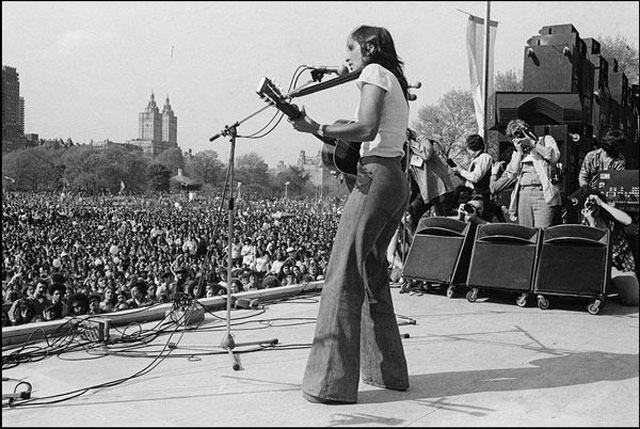The black-and-white photograph captures an outdoor concert likely from the 1970s. At the center of the image, a woman stands on a large stage, performing with an acoustic guitar in hand and singing or speaking into a microphone. She is dressed in bell-bottoms and a fitted light-colored shirt with short, flowy sleeves, her dark hair pulled back by a headband or careful securing. Surrounding her, particularly to the right, are several photographers capturing the moment. To the left and stretching into the background are tens of thousands of concert-goers, their presence forming a massive crowd that blends into distant buildings, hinting that this could be taking place in an iconic urban park like Central Park, New York City. The sky above is visible, with scattered clouds adding depth to the scene, while numerous wires snake across the stage floor, contributing to the technical setup of this professionally photographed event.